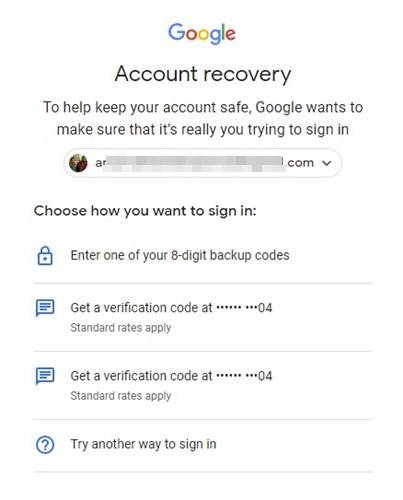The image depicts a Google Account Recovery page, designed to help users secure their accounts. The page has a clean, white background with "Google" displayed prominently at the top in the familiar blue, red, yellow, and green logo. Below the logo, the text is primarily in black. 

The largest text on the page reads "Account Recovery." Immediately beneath this title, there is a message that states, "To help keep your account safe, Google wants to make sure that it's really you trying to sign in." 

Following the message is a drop-down section containing the user's partially blurred name and information. A profile picture is also present, though the details of the picture are indistinguishable. 

The next section prompts the user to choose a method for verifying their identity, the first option being, "Enter one of your 8-digit backup codes." There is a text line for entering the code, followed by an option, "Get verification code at [number]…04," indicating the last digits of the linked phone number. The phrase "standard rates apply" is mentioned twice in smaller text.

Below these verification options are fields that resemble text boxes and a question mark icon in a circle, indicating more ways to sign in. These icons are rendered in blue, complementing the black, white, and gray color scheme of the rest of the page, save for the vibrant Google logo at the top.